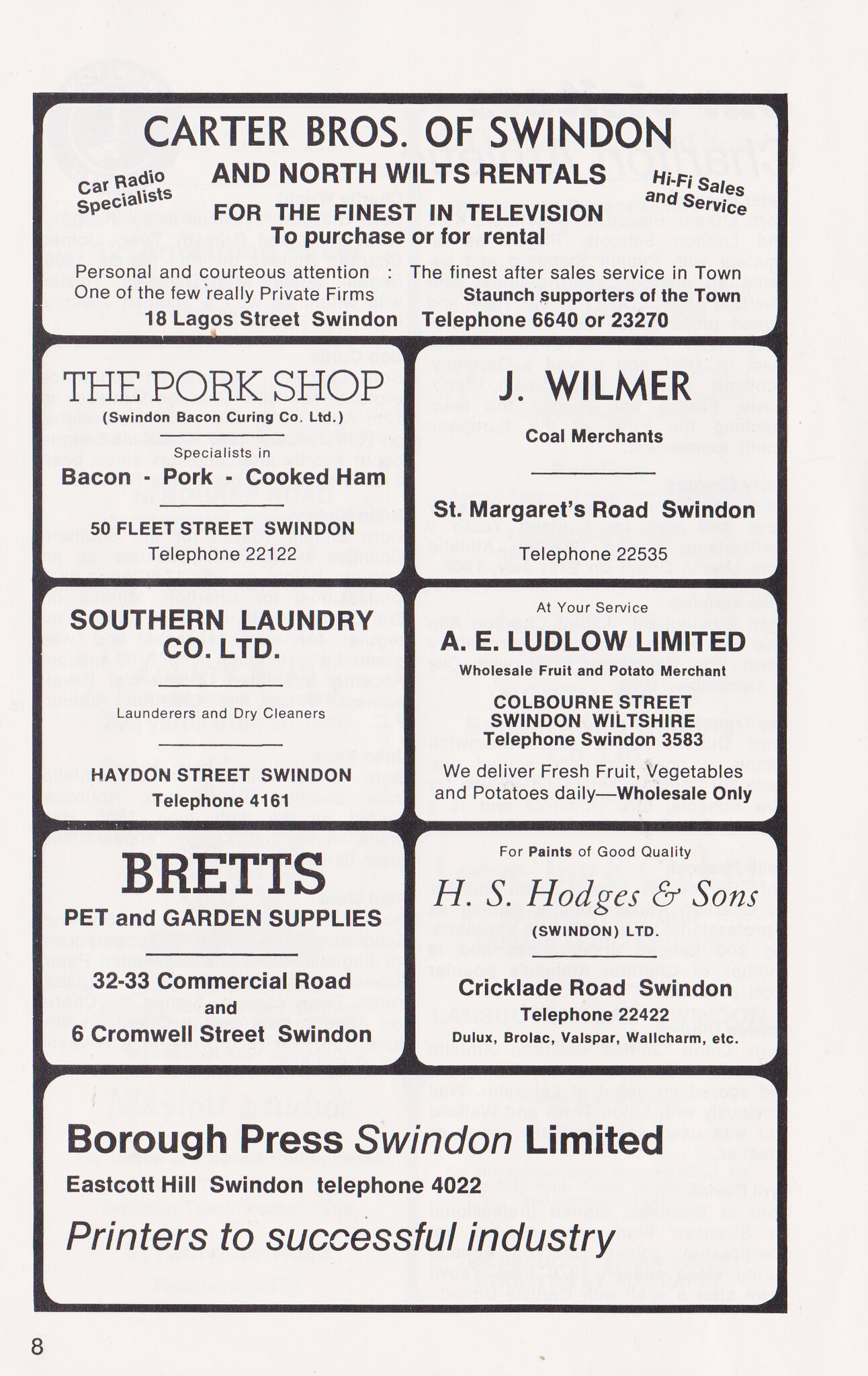This image showcases a collection of eight black-and-white advertisements for various businesses, seemingly from an older newspaper page. The top advertisement is for Karcher Brothers of Swindon and North Wilts Rentals, highlighting their offerings in television sales and rentals, hi-fi sales and services, and car radio specialization. They pride themselves on personal and courteous attention, being one of the few really private firms, boasting the finest after-sales service in town, and are staunch supporters of the community. Their address is 18 Lagos Street, Swindon, with telephone numbers 6640 and 23270.

Directly below are two ads side by side: on the left, The Pork Shop, specializing in bacon, pork, and cooked ham, located at 50 Fleet Street, Swindon, with telephone number 22122; on the right, J. Wilmer Coal Merchant, located at St. Margaret's Road, Swindon, with telephone number 22535.

Further down, another pair of side-by-side ads feature Southern Laundry Co. Ltd., offering laundry and dry cleaning services, located on Hayden Street, Swindon, with telephone number 4161, and A.E. Ludlow Limited, a wholesale fruit and potato merchant from Colborne Street, Swindon, Wiltshire, with telephone number 3583. They deliver fresh produce daily on a wholesale basis.

The next set of advertisements includes Brett’s Pet and Garden Supplies, situated at 32-33 Commercial Road and 6 Cromwell Street, Swindon, and H.S. Hodges & Sons, offering quality paints, located on Crick Laid Road, Swindon, with telephone number 22422. They carry brands like Dulux, Brolac, Valspar, and Well Charm.

At the very bottom is the final ad for Borough Press Swindon Limited, printers to successful industry, located at Eastcott Hill, Swindon, with telephone number 4022.